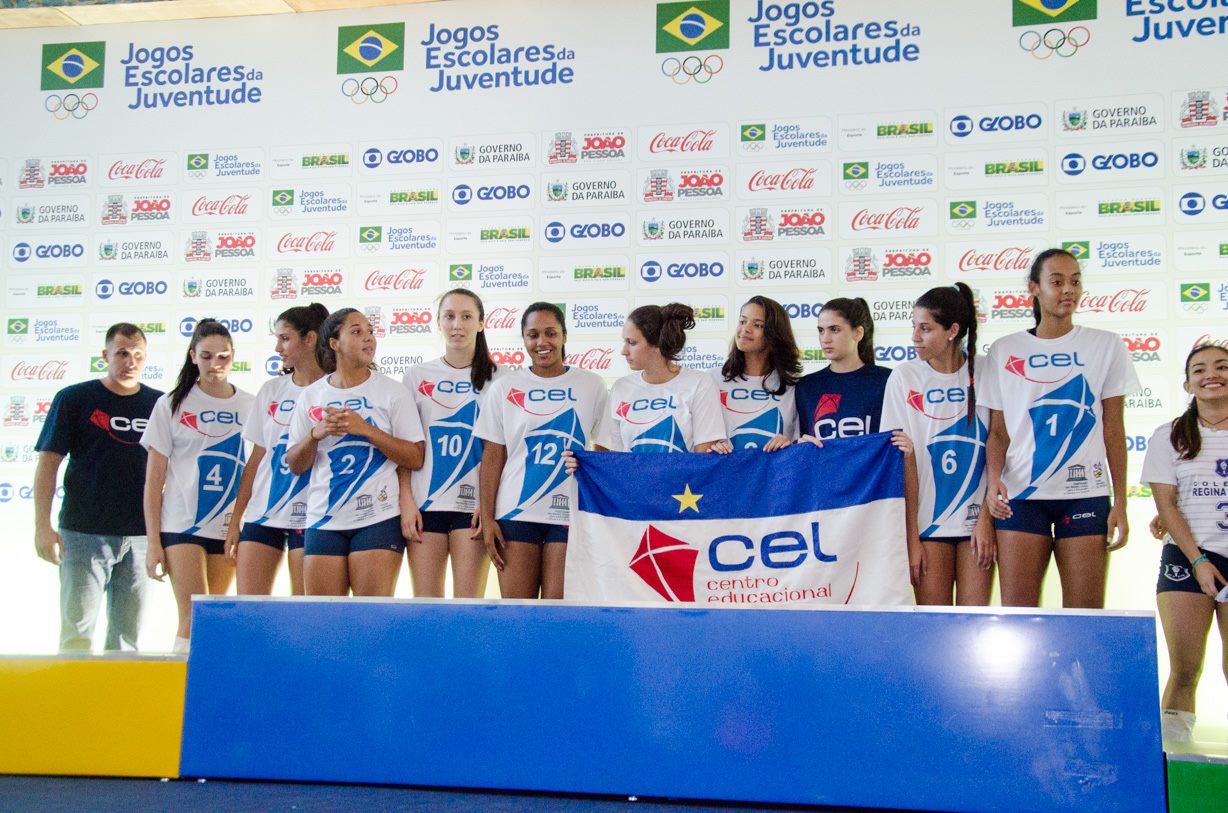In the image, a color, landscape-oriented photograph, a group of 12 teenage girls is depicted standing on a stage, apparently at an awards ceremony for a sports event. The girls, arranged from the far left to the right, wear matching white jerseys featuring a blue kite logo with individual numbers ranging from 1 to 12. They are also dressed in dark sports shorts with their hair styled in either ponytails or braids. Three girls at the center hold a banner displaying a blue stripe at the top, a yellow star, and a white section below with a red kite and the text "C-E-L" in blue, followed by "Centro Educational" in red. 

To the far left of the group stands the only man in the scene, presumably a coach, dressed in blue jeans and a black shirt with the same "C-E-L" and red kite logo. He appears to be in his mid-thirties with short hair. Behind the group is a backdrop filled with various advertisements and logos, including the Olympic rings, and the repeated text "Jogos Escolares da Juventude," amidst sponsors such as Coca-Cola and Jojo. Additionally, the stage has a distinct blue wall up to knee height, flanked by a shorter yellow fence to the left and a green structure to the right.